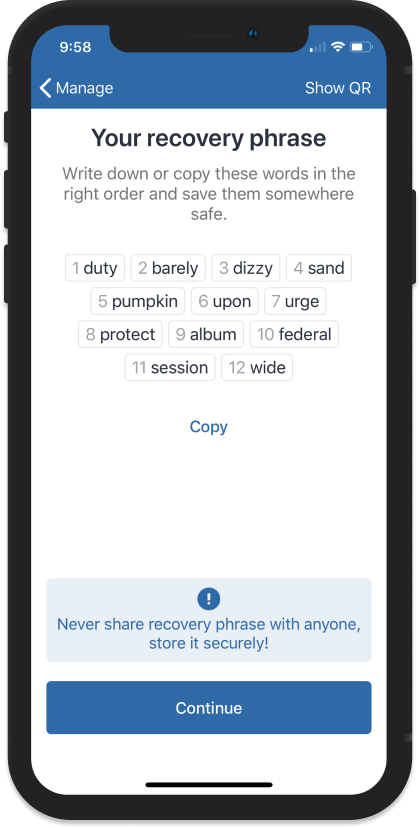The simulated image showcases the screen and outer frame of a smartphone. The solid black frame includes visible details such as the power button, volume button, and a small lighter blue reflection in the upper right-hand corner indicating a camera lens, along with a tiny indent for the speaker.

On the phone screen, the top half features a bright blue border with white text. The time in the upper left-hand corner reads 9:58, and the upper right-hand corner displays three icons: a Wi-Fi icon with three bars (indicating low signal), a signal bars icon with one bar illuminated, and a battery icon showing more than half charge. Below the time, white text reads "Manage" with a left-facing arrow, and "Show QR" appears beneath the battery icon.

The main area of the screen has a white background with black text. The first line reads "Your Recovery Phrase" followed by gray text instructing users to "Write down or copy these words in the right order and save them somewhere safe." Below this, there are twelve numbered tabs, each displaying a word: Duty, Barely, Dizzy, Sand, Pumpkin, Upon, Urge, Protect, Album, Federal, Session, and Wide. Beneath these tabs is bright blue text labeled "Copy."

At the bottom, a light blue rectangular box contains bright blue text advising users to "Never share recovery phrase with anyone. Store it securely." Above this warning is a blue circular icon with a white exclamation point in the center. Finally, at the very bottom of the screen, there is a large rectangular blue button with the word "Continue" in white text at its center.